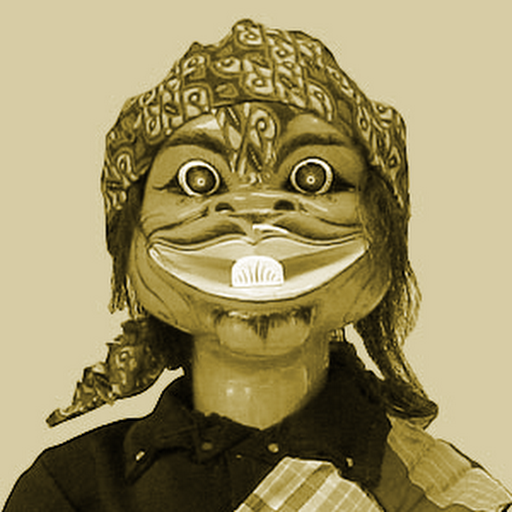The image depicts a humanoid carved doll with a monstrous appearance, visible from the shoulders upwards. The doll is clad in a black collared button-up shirt with clear buttons fastened all the way up, draped over its shoulders with a plaid scarf or shawl. Its face and neck are intricately carved from wood, featuring large round white eyes with black circles in them, giving it a haunting expression. The face showcases highly stylized shadowing and a wide, white-painted smile that stretches across its mouth. The nose is rounded with forward-facing nostrils and there seems to be a possible goatee at the bottom of the face. A dark-colored headband adorned with various circle designs sits atop its head. Long strands of hair cascade down the left and right sides of the face. The entire image is tinged with muted, possibly monochromatic colors such as gray, brown, black, and off-white, contributing to its eerie yet artistic presence. While well-centered, the doll's unsettling yet artful composition could be suited for a scare house or a historical display, evoking curiosity and a sense of mystery.